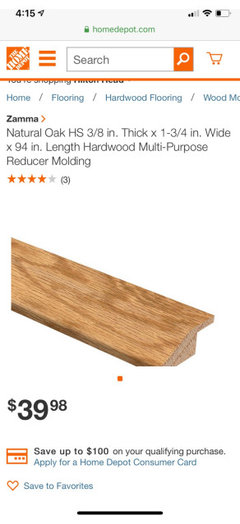The screenshot displays a cell phone's interface with a grey background at the top. On the upper left side, in black text, it reads "415." To the right of this text, the GPS icon is visible, followed by a blank grey space. The icons for cell phone coverage, Wi-Fi, and battery are also visible on the top right side. Below this, an address bar shows the URL "HomeDepot.com" in grey text. 

Immediately underneath the address bar, on the left side, the Home Depot logo is prominently displayed. The logo consists of an orange square with "Home Depot" written in white. Adjacent to the logo, three horizontal bars are shown, representing a menu. There is a search bar with a magnifying glass icon, and a shopping cart icon next to it.

Beneath this, blue text indicates the webpage hierarchy: "Home / Flooring / Hardwood Flooring / Wood Moulding." Below this, in black text, the product name "Zamma" (spelled Z-A-M-M-A) is displayed, followed by grey text describing the product: "natural oak HS 3/8 inch thick X 1-3/4 inch wide X 94 inch length hardwood multipurpose reducer moulding." This product has a rating of 4 out of 5 orange stars, based on three reviews.

To the right, a small image of a light tan natural wood piece is shown. Below this image, the price is listed in black text as "$39.98." Further down, an orange credit card icon is displayed alongside a black text offering: "Save up to $100 on a qualifying purchase. Apply for a Home Depot consumer card."

On the left side, there is an orange heart icon that is not filled in, and in grey text, it says "Save to favorites." Finally, at the very bottom of the screen, a small black bar contains additional cell phone interface elements.